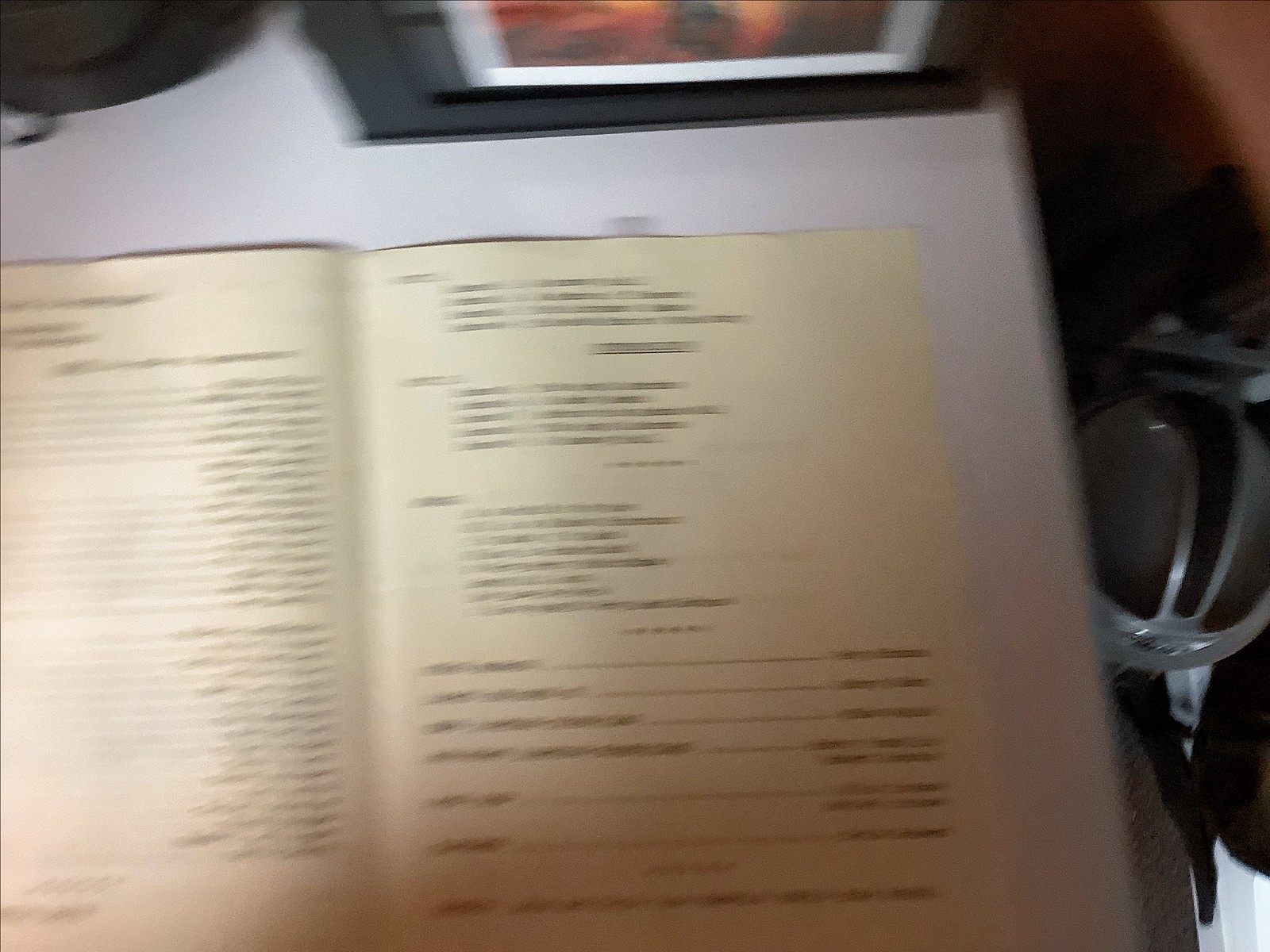This landscape-style image, taken with a camera, shows a blurry open book with two pages in a cream off-white color. The pages are adorned with blurry, unreadable black text, which might suggest it is a cookbook. The book is prominently displayed on a white table occupying most of the left and central part of the image. A black picture frame with a red and orange blurred picture inside rests on top of the table. The right side shows a blurry red background. To the left of the book, there is a partly visible grey and black trash can or bin, while the bottom right features indistinct white objects. The overall image has a mix of colors, with blurry and partly indiscernible elements that add to its intriguing, unfocused nature.